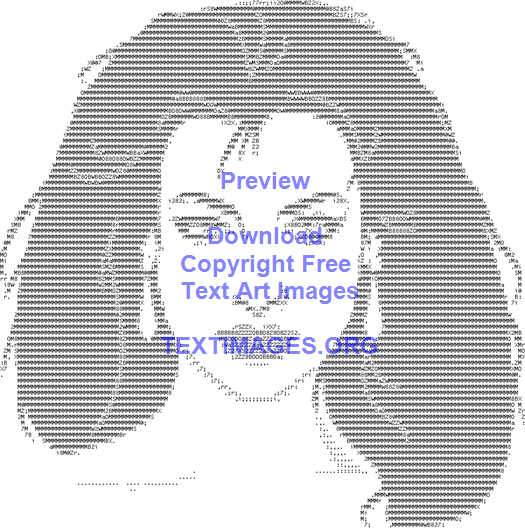This preview image from textimages.org showcases a pixelated, text art depiction of a woman's face and hair against a completely white background. The pixelation gives her long black and white hair a distinct, stylized appearance as it cascades down to her shoulders. She faces forward, allowing for a clear view of her eyes, nose, and mouth, as well as her neck and shoulders. She is adorned with white drop earrings that add a touch of elegance to the minimalist art style. Despite the overlaid blue font advertisment for textimages.org, which partially covers her face, the woman's features remain discernible and the overall preview provides a clear example of the kind of images available for download from the site.